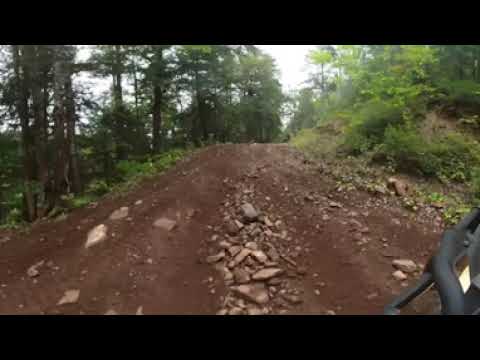This image captures a cyclist's viewpoint traveling along a naturally formed dirt path in a forest. The dark brown path, scattered with rocks and pebbles, winds through a dense array of tall, green trees and bushes that flank both sides. The sky, visible in the top middle and top left of the image, appears bright and white, suggesting a clear and sunny day. The low-resolution picture seems to have been taken from a helmet camera, as evidenced by the black framing at the top and bottom and a possible part of a bicycle visible in the bottom right corner. The rugged, rocky terrain could indicate a challenging ride for the cyclist.